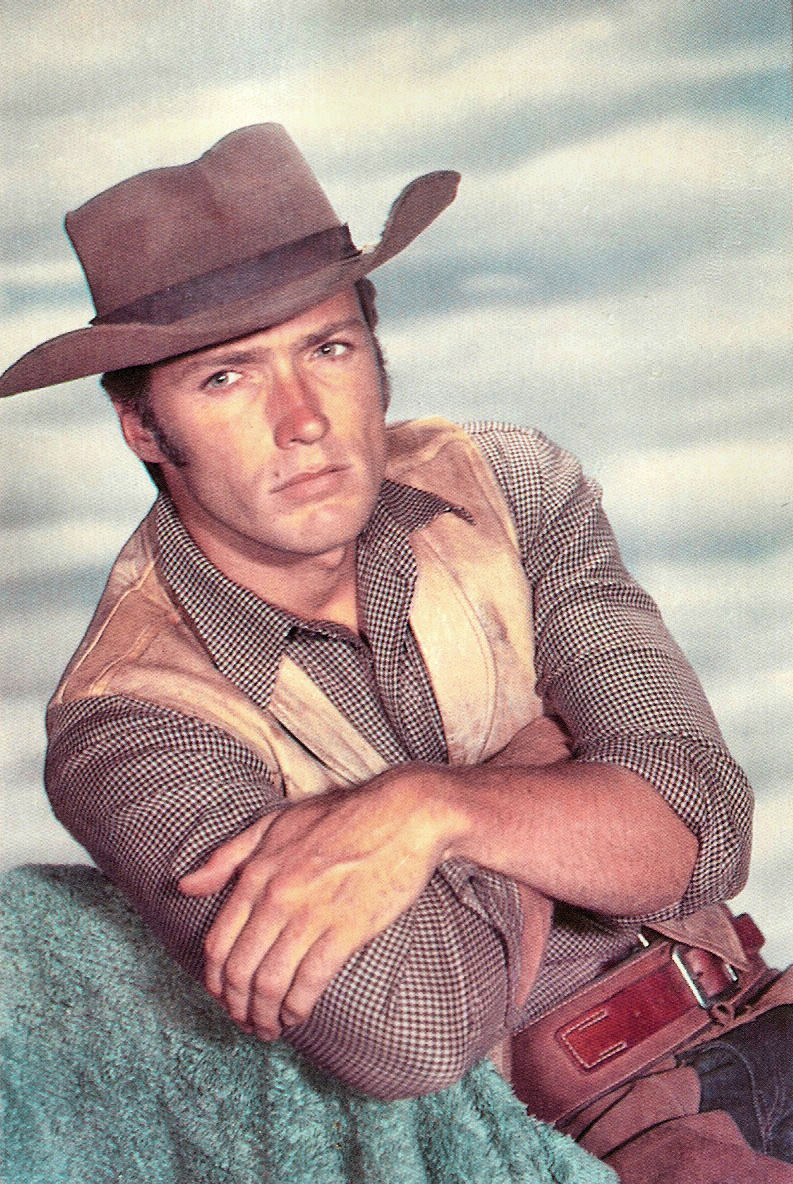In this color-restored photograph from the television western "Rawhide," a young Clint Eastwood poses with a serious expression. He leans against a green blanket-covered object, initially appearing like a rock, with arms crossed. The backdrop suggests clouds in an overcast sky. Clint is dressed in a classic cowboy outfit, featuring a light brown cowboy hat with a darker band, a leather vest over a checkered button-down shirt with white squares and black stripes, and dark blue pants with brown suede chaps. A gun belt, complementing his attire, adds to his rugged look, and his short light brown hair and greenish eyes are clearly visible. The pants sport a built-in buckle and the chaps feature a red and black leather vest. Additionally, there's a distinctive mole on the left side above his upper lip.